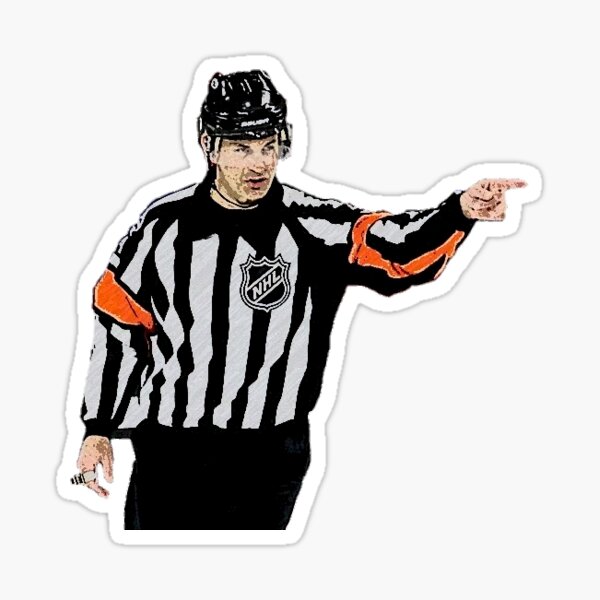This image appears to be a stylized sticker or magnet of an NHL referee, illustrated in a cartoon-like manner. The referee is a white male, dressed in a traditional black and white vertically striped shirt, featuring an NHL crest prominently on the chest. The stripes on the shirt are black and light gray, with distinct orange horizontal stripes encircling the sleeves. He is equipped with a shiny black helmet and a clear plastic face shield. His facial features include light brown splotches, suggesting the image may be slightly blurry or of low quality. The referee is depicted from around the thigh upwards, wearing black pants. The right arm is extended outward with his index finger pointing to the right, while his left arm rests at his side holding a whistle. The background of the image is a light gray, enhancing the contrast and making the character stand out.